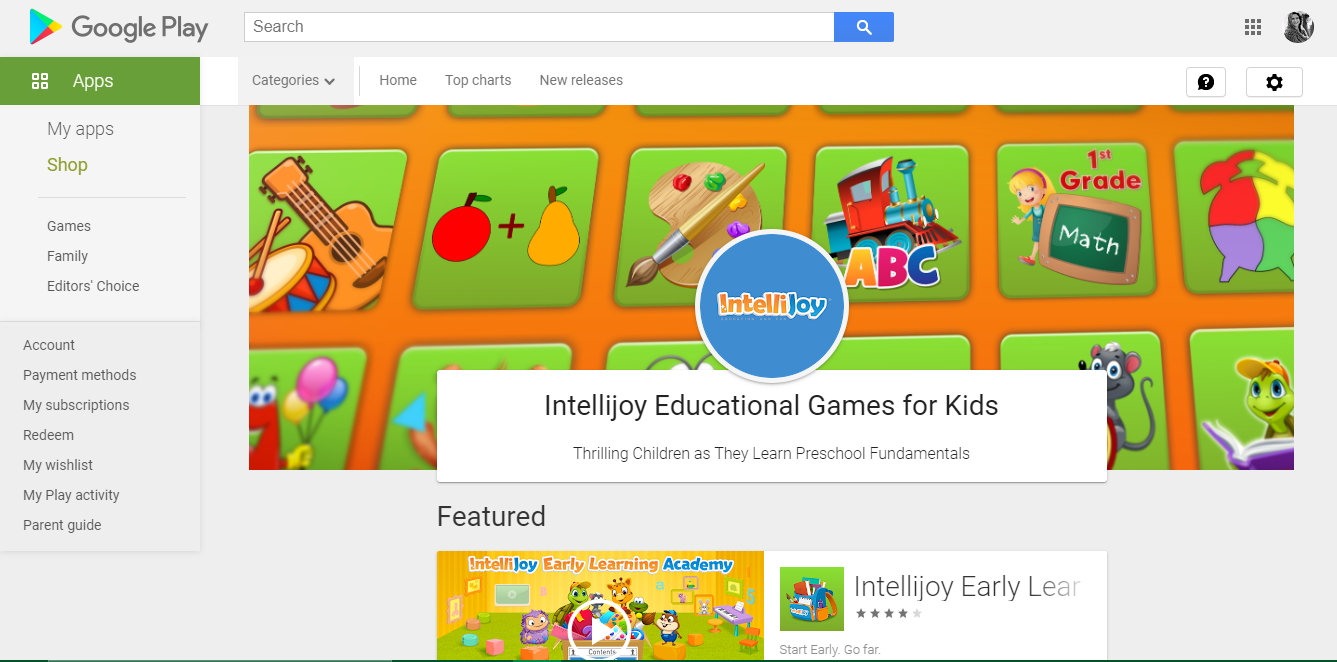In the upper left corner, there is a right-pointing arrow fashioned as a triangle, featuring the colors blue, red, and yellow. Next to it, the words "Google Play" are displayed. Below this, in a green rectangle, is the label "Apps," accompanied by four small white squares to the left of the word.

Underneath the rectangle, a menu lists the following options: My Apps, Shop (highlighted in green), Games, Family, Editor's Choice, Account, Payment Methods, My Subscriptions, Redeem, My Wish List, My Play Activity, and Parent Guide.

The center of the page is vibrant with colorful squares, suggesting a child-friendly web page design. Each square contains engaging images: a drum and a guitar, an apple and a pear, a paintbrush with a palette, ABC and a train in a green square, first-grade math featuring a smiling child figure, and lively colors of red, yellow, purple, and green.

At the center of this layout is a blue circle with the text "Intel Joy." Beneath this circle, the words "Intel Joy - Educational Games for Kids" are prominently displayed.